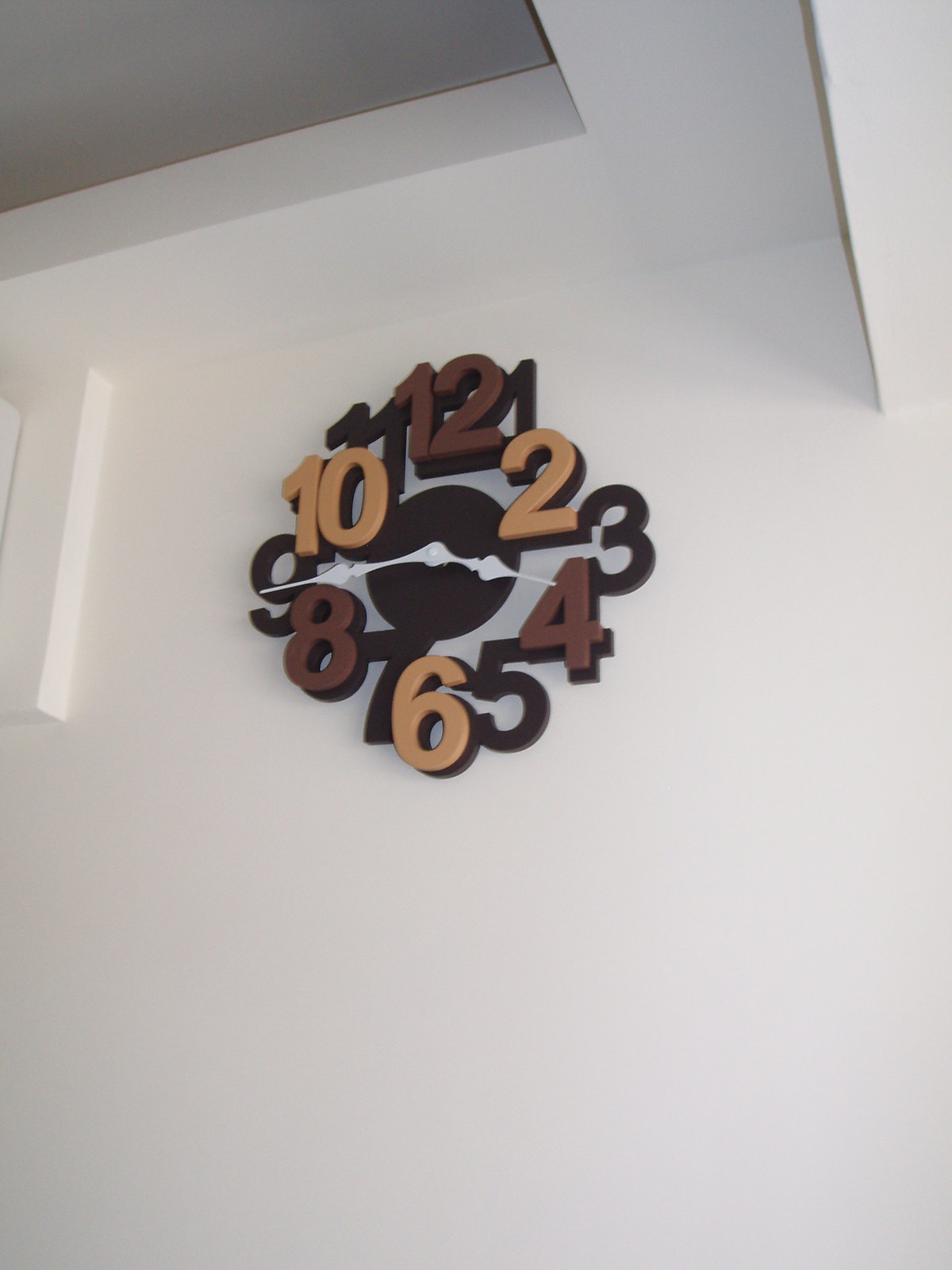This vertical rectangular photograph captures a minimalist interior view, prominently featuring a white wall with a matching white ceiling. At the very top left, the ceiling transitions to a dark gray recessed area. A rectangular trim separates the ceiling from the wall. Centrally positioned high up on the wall, towards the upper right-hand corner in the context of the image, hangs a round, brown clock with slightly raised numbers that provide a 3D effect. The clock face includes alternating colored numbers: dark brown for odd numbers (1, 3, 5, 7, 9, 11) and a combination of medium, light, and yellowish-brown for even numbers (2, 4, 6, 8, 10, 12). The clock hands are white, and the time displayed is approximately 4:42, indicated by the small hand pointing to the 4 and the big hand situated between the 8 and the 9.